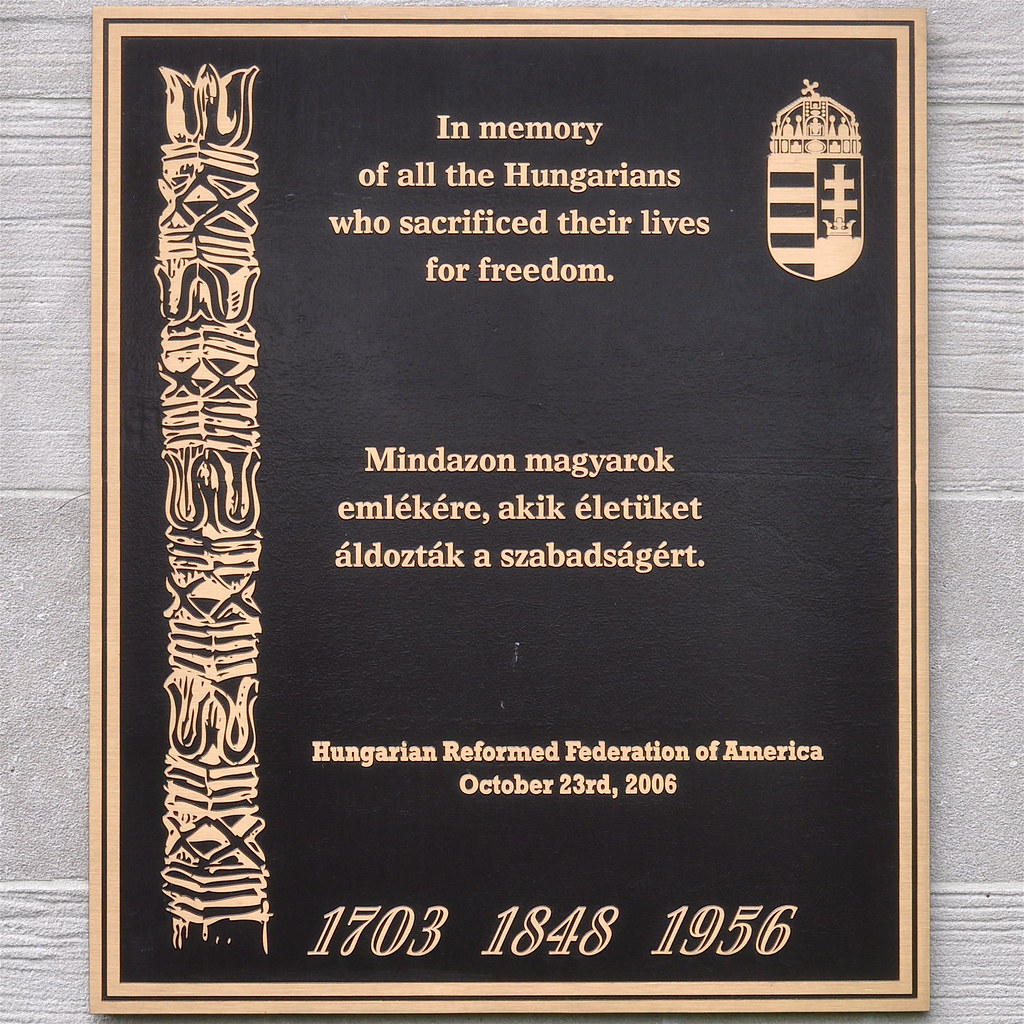This image depicts a memorial plaque mounted on a gray concrete wall with visible striations. The plaque itself features a black background framed by a gold border, with an additional gold decorative column running the full length of the left-hand side. The top right corner of the plaque showcases a gold crest with intricate black detailing. The primary inscription, written in gold letters, reads, "In memory of all the Hungarians who sacrificed their lives for freedom." Beneath it, there is a section in Hungarian: "Mindazon Magyarok Imlikeri Akik Elituket Aldozdak Azabadsagaret." Following this, the text notes, "Hungarian Reformed Federation of America, October 23rd, 2006." At the very bottom of the plaque, three significant years are listed: 1703, 1848, and 1956.